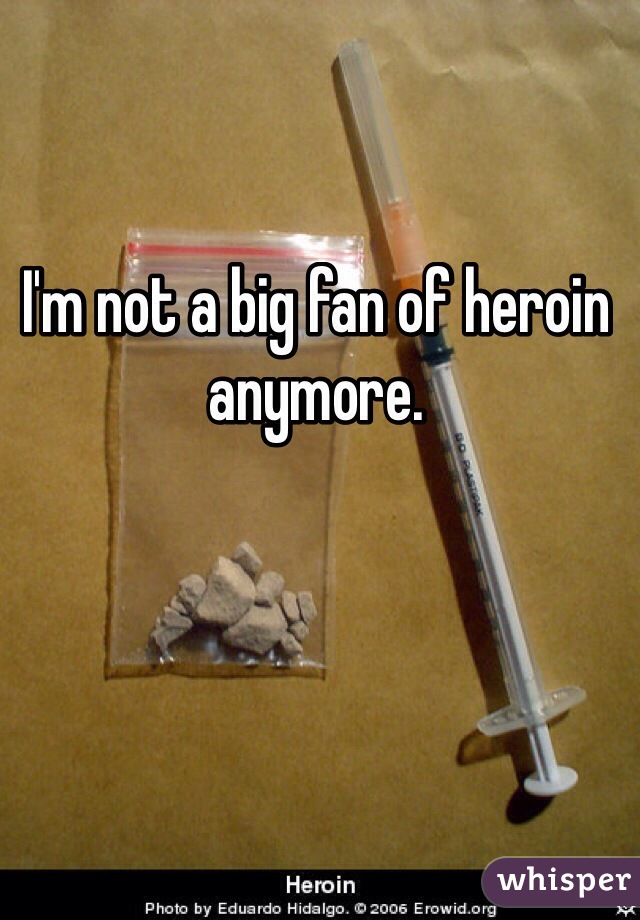This detailed image, reminiscent of a meme, captures a stark scene of drug paraphernalia: a thin white syringe, capped with a clear plastic cover that reveals an orange and black needle, lies next to a small Ziploc bag filled with varying sizes and shapes of gray rocks, likely chunks of heroin. The items rest on a brown surface that resembles a paper bag, enhancing the raw and gritty context of the image. Across the center of the image, white text with a black outline states, "I'm not a big fan of heroin anymore." The bottom of the image features a black horizontal bar bearing the words "heroin, photo by Eduardo Hidalgo, 2008, eroid.org," while a small purple banner in the lower right corner simply reads, "whisper." This composition collectively suggests a powerful narrative of overcoming addiction, marked by minimal yet striking color contrasts.